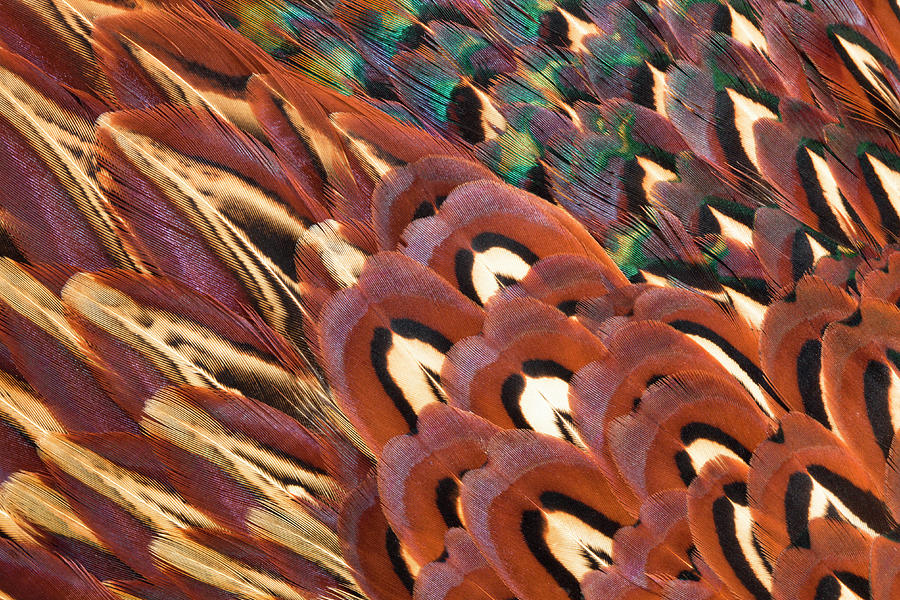This detailed close-up painting showcases an eclectic array of intricately detailed feathers, layered and overlapping in a dynamic composition that flows diagonally from the lower right to the upper left. The feathers vary greatly in shape and color, creating a rich and textured visual experience. Prominent among them are reddish-brown feathers with white interiors and black outlines. These are seamlessly interwoven with peacock-like feathers in the top right, boasting a palette of teals, blues, and purples with brown centers. Some feathers display a gradient of orange to burnt sienna, with lighter tan centers and subtle black detailing, while other feathers feature elongated stripes of red and beige punctuated by black accents. Each feather is meticulously rendered, capturing individual hairs and the delicate thin elements that constitute their structure, suggesting a close-up view of a larger, possibly zoomed-in section of a bird’s plumage.